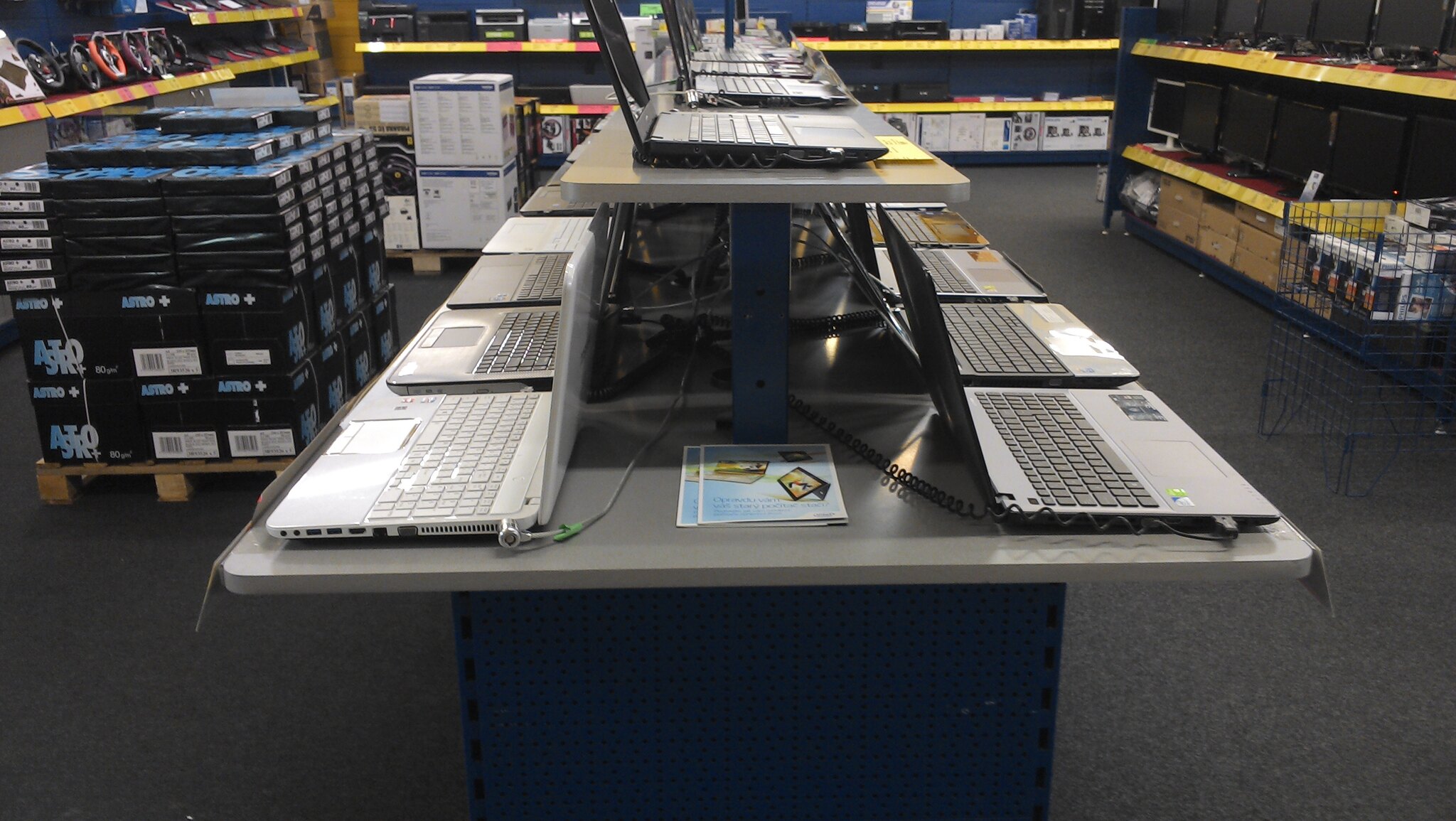This detailed photograph captures the bustling environment of an electronics store, likely a place like Best Buy. At the center of the image, a long rectangular table showcases an array of laptops. These laptops come in various colors and are neatly aligned in a row, with the screens open to reveal their keyboards. On the left frontside of the table, a white laptop with matching keys is visible, while a black laptop with black keys stands out on the right frontside. Above this main table, an additional raised platform continues the display with more laptops securely attached by security cords.

The side view perspective offers a comprehensive look down the lineup of laptops, highlighting their different colors and features. In the background, shelves are packed with diverse electronics, including printers and computer towers, with bright yellow pricing tape marking the costs. To the left, a pallet stacked with packages of printer paper is visible, while to the right, TV or computer monitors are exhibited on shelves. Further right, a blue wire basket container holds Polaroid cartridges.

Overall, the photograph vividly portrays the organized yet busy scene of an electronics store, emphasizing the central table laden with a variety of laptops amidst an abundance of related electronic products.